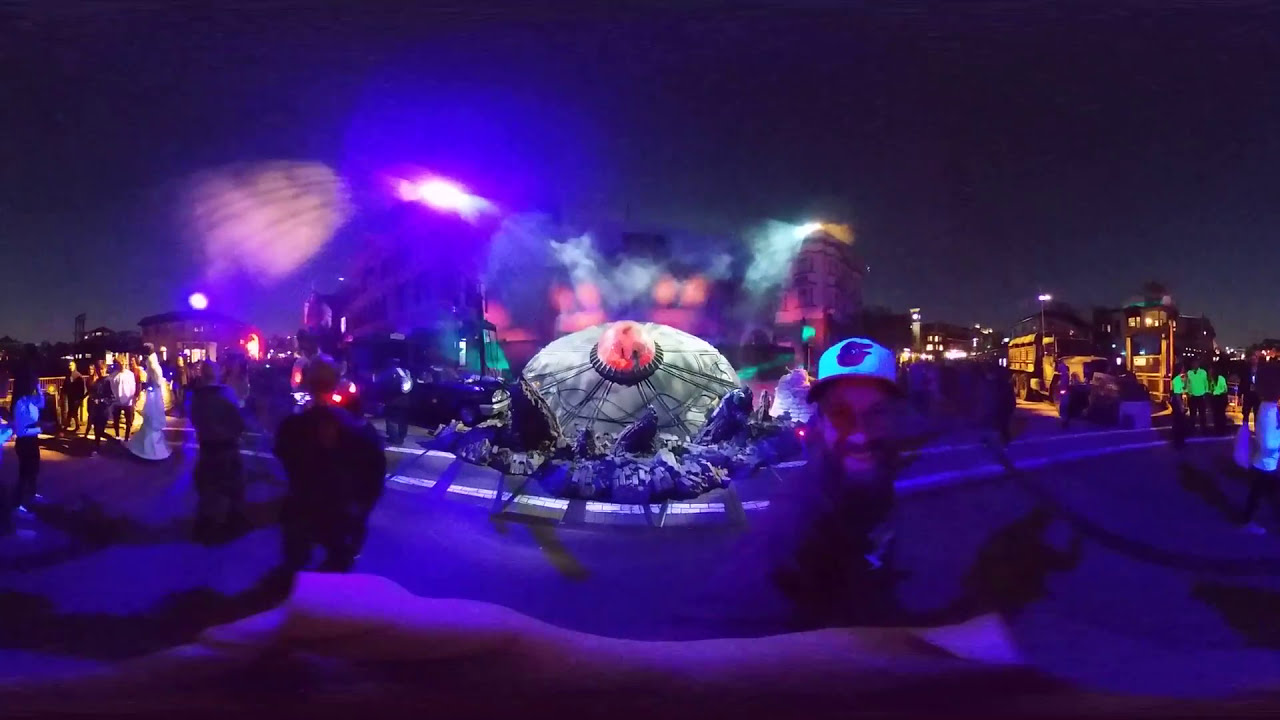The image captures a vibrant nighttime scene, bathed predominantly in blue light. At the center of the composition is a captivating display resembling a crashed UFO, with a circular, gray, and round shape featuring a prominent red orb on top. Jagged rocks surround the base of this UFO-like structure, adding to the dramatic visual. Smoky effects and various colored lights, including pinks, greens, yellows, and purples, enhance the atmosphere, suggesting a theatrical or amusement park setting. Surrounding this central object are numerous people, intrigued by the spectacle. In the background, lit-up buildings further contribute to the lively ambiance. On the right side of the image, there are military vehicles or trucks parked, seeming to add an element of curiosity and intrigue to the scene. One man stands out, smiling directly at the camera and wearing a white and red baseball cap, providing a personal touch to this dynamic and detailed photograph.